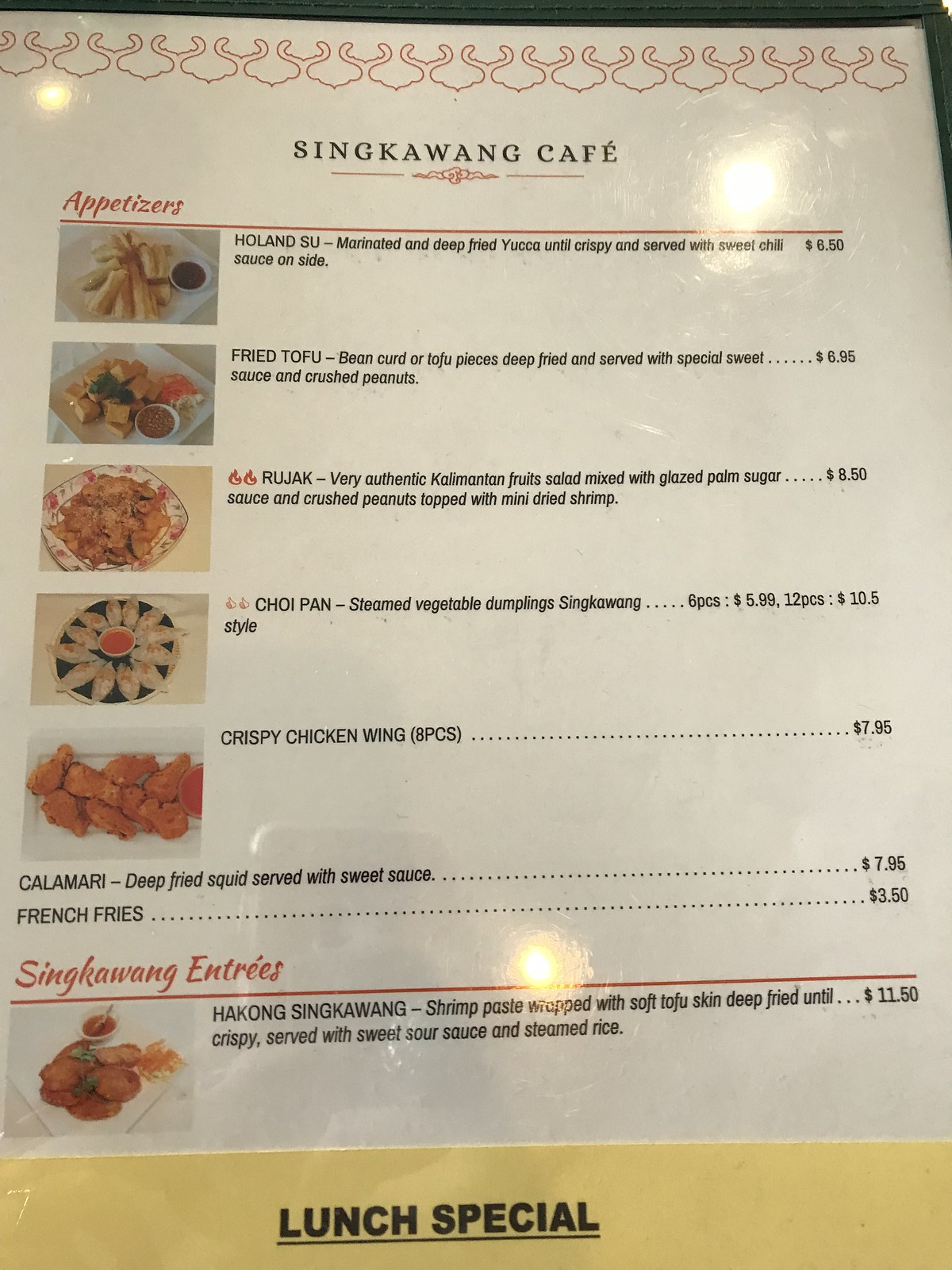This photograph features a detailed menu from "Sang Kwang Café," showcasing a variety of enticing food items on a white background. 

At the top of the menu, in bold black all-caps typography, it reads "SANG KWANG CAFE," with the letter 'E' adorned with an accent. Above this title is a decorative red design, resembling an abstract pattern of horns and bells in a continuous undulating line.

Below the café's name, in red ink, the section titled 'Appetizers' is prominently displayed on the left side with a horizontal line extending rightwards. The menu lists five appetizers, each accompanied by a thumbnail image on the left. The listed items are:

1. **Holland Sous** - Price not mentioned.
2. **Fried Tofu** - Described as bean curd pieces deep-fried and served with special sweet sauce and crushed peanuts. Priced at $6.95.
3. **Rujak** - Marked with two fiery symbols indicating spiciness.
4. **Choy Pan** - No description provided.
5. **Crispy Chicken Wings (8 pieces)** - Priced at $7.95.

Additionally, two more appetizers without images are listed towards the bottom:

6. **Calamari** - Described as deep-fried squid served with sweet sauce. Priced at $7.95.
7. **French Fries** - Priced at $3.50.

Underneath the appetizers section, a new section titled "Sang Kwang Entrées" appears in red. The visible entrée is:

- **Hakong Sing Kwang** - Accompanied by a detailed two-line description, priced at $11.50.

At the very bottom of the menu, a yellow strip occupying roughly 10% of the page highlights the phrase "Lunch Special" in bold black text. Unfortunately, the specifics of the lunch specials are cut off from the view.

This well-organized menu, though partially visible, provides a glimpse into the diverse offerings of Sang Kwang Café, capturing the appetite with detailed descriptions and vivid imagery.